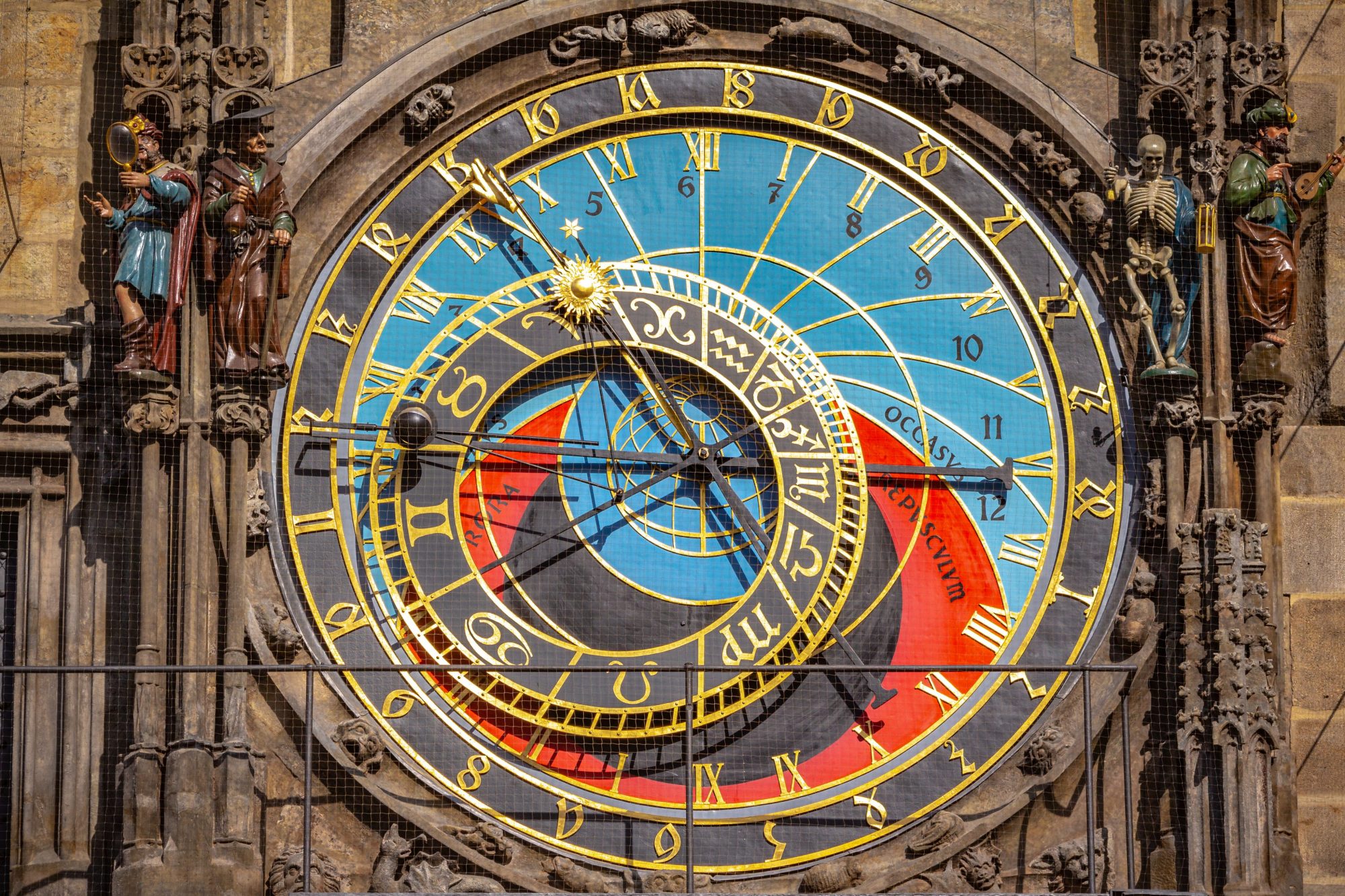This detailed close-up photograph showcases an elaborate, multicolored medieval-style clock face mounted on the side of an outdoor building, likely a clock tower, captured during the daytime. The clock is flanked by stone pillars adorned with statues. On the right pillar stands a skeleton statue, alongside a figure in a green jacket and brown robe, wearing a turban and holding a lute. The left pillar features a statue of a man in a cap resembling a graduate's, dressed in a brown robe and holding a cane, next to another figure in an orange robe with outstretched hands.

The clock's face is intricate, with multiple bands and dials. It has an outer black ring bordered in gold, featuring peculiar rune-like symbols. Inside this, there's a ring displaying Roman numerals from I to XII in gold, interlaid with standard numerals 1 through 12 in blue. Another smaller circle depicts various zodiac signs, indicating potential astrological significance. The face includes a prominent red half-circle band towards the bottom with the letters "OCCASV, EPVSCVIVM" and "RORA."

The clock is also marked with numbers ranging from 1 to 24, suggesting it might function as a 24-hour timepiece. These numbers are displayed prominently around the edge, with a distinctive design for the number 24 that appears as a 2 followed by a ribbon-like figure.

The clock hands differ in design: the longest hand has a black dot, the second longest features a golden sun, and the shortest lacks any distinct marking. The longest hand points to nine, the second longest is between nine and ten, and the shortest points to ten. The clock face's colors include shades of blue, red, gold, and black, contributing to its visually striking appearance.